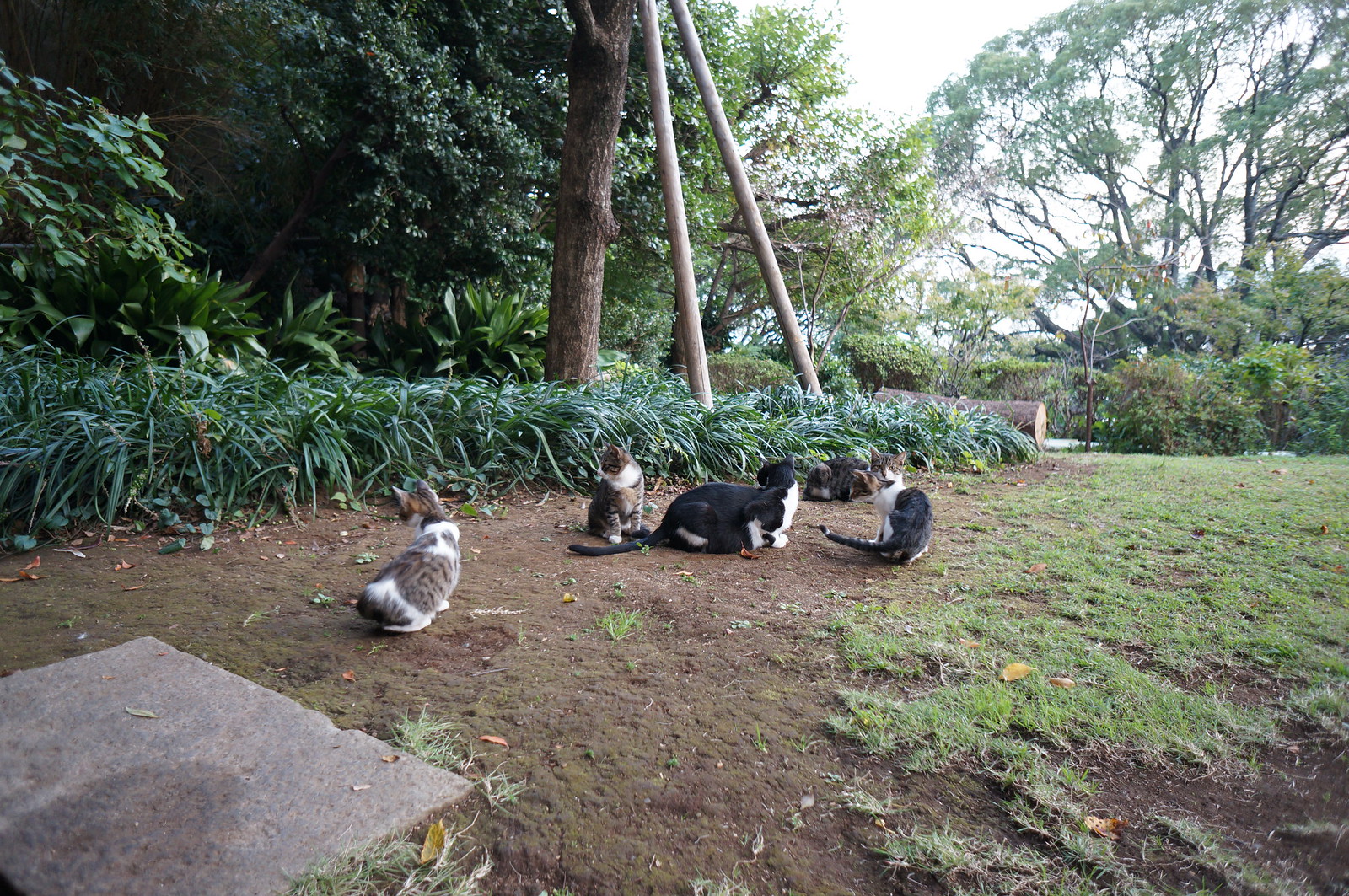In this photograph set in what seems to be a backyard, five cats of different colors and ages—ranging from black and white to brown tabby and white—are either sitting or walking on a patch of bare dirt. The area they are in is bordered by sparse grass on the right side and more robust greenery on the left, which includes small shrubs, larger bushes, and tall trees with thick trunks, supported by posts. Among these cats, one situated on the leftmost side appears to be missing a tail. A small concrete block resembling a step is positioned in the lower left corner of the image, adding to the backyard feel. The cats, short-haired and possibly feral, all have their attention directed in different ways. Three of them are looking over their shoulders towards the left, where the dense foliage lies, while one is gazing directly at the camera. The background sky, visible in the upper right corner, is bright white, providing a stark contrast to the rich greenery and earthy tones of the setting.